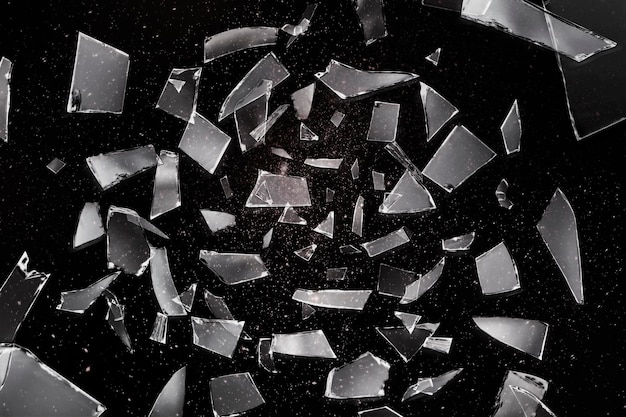This black and white image vividly depicts the vastness of space, characterized by a solid black background filled with dispersed small white specks that resemble stars. Dominating the scene are numerous shards of shattered glass, each broken into various sizes and sharp-edged shapes such as squares, rectangles, and irregular forms. The fragments float amidst the stars, some even reduced to the tiniest powders, sparking the illusion of a cosmic explosion. This striking imagery, reminiscent of the iconic Twilight Zone intro, showcases glass pieces seemingly suspended in the endless cold of space, creating a mesmerizing contrast between the chaotic debris and the serene, distant galaxy.